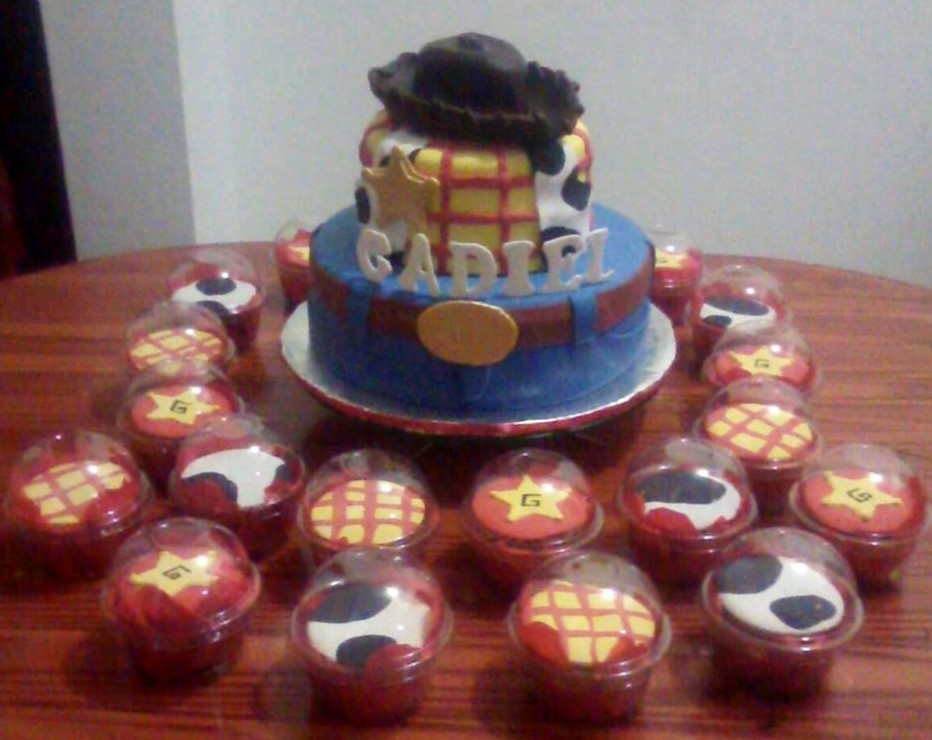The slightly blurry image shows a two-tiered, Toy Story-themed cake on a round dark wood table inside a dimly lit room with white walls. The bottom tier of the cake represents blue denim pants with a brown belt and a gold belt buckle. The second tier resembles a yellow and red checkered shirt adorned with a white fondant cowhide vest and a gold sheriff's star badge, completing the look of Woody from Toy Story. At the top sits a dark brown fondant cowboy hat. The name "GADIEL," spelled out in white frosted letters, stands out prominently on the blue part of the cake. Surrounding the cake are at least 17 individually packaged cupcakes in clear dome containers, each featuring the same thematic designs: red and yellow plaid, black and white cowhide, and sheriff stars with the number six. The table is placed near a corner with an opening to another room visible in the left-hand corner of the photo.